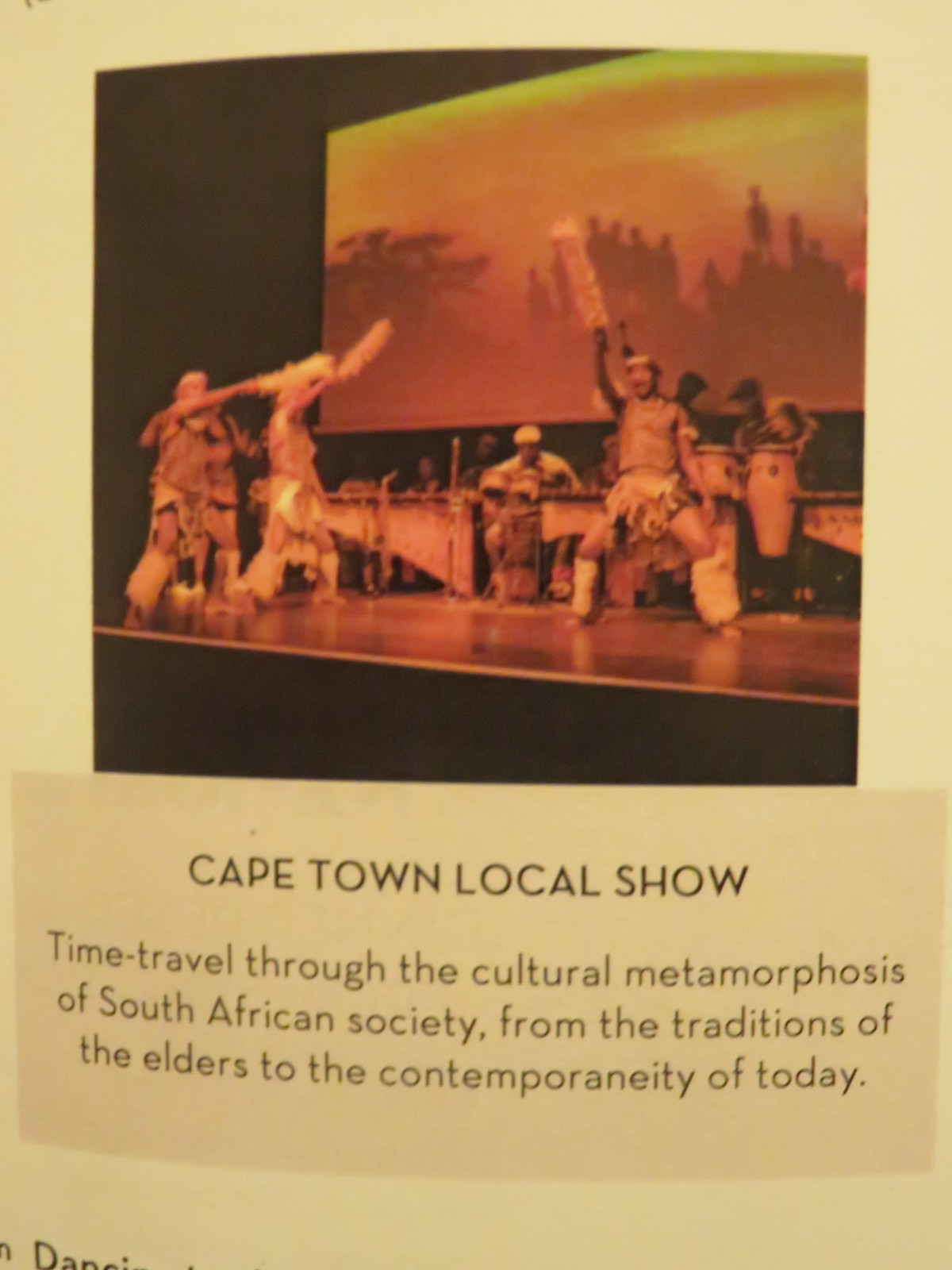The image captures a photograph of a page, possibly from a museum exhibit, flyer, or pamphlet. The top portion of this page displays a photograph of a Cape Town local show. In the photograph, at least three performers are on stage, engaging in what appears to be a traditional African dance. They are adorned in vibrant, African tribal attire, adding authenticity to the performance. Behind them, several musicians play traditional instruments, contributing to the cultural atmosphere. There is a projector screen in the background displaying an African scenery bathed in hues of orange and yellow. Below the photograph, text describes the exhibit as "Cape Town local show: Time Travel through the Cultural Metamorphosis of South African Society from the Traditions of the Elders to the Contemporaneity of Today." This detailed description offers a glimpse into the rich, evolving culture of South African society.